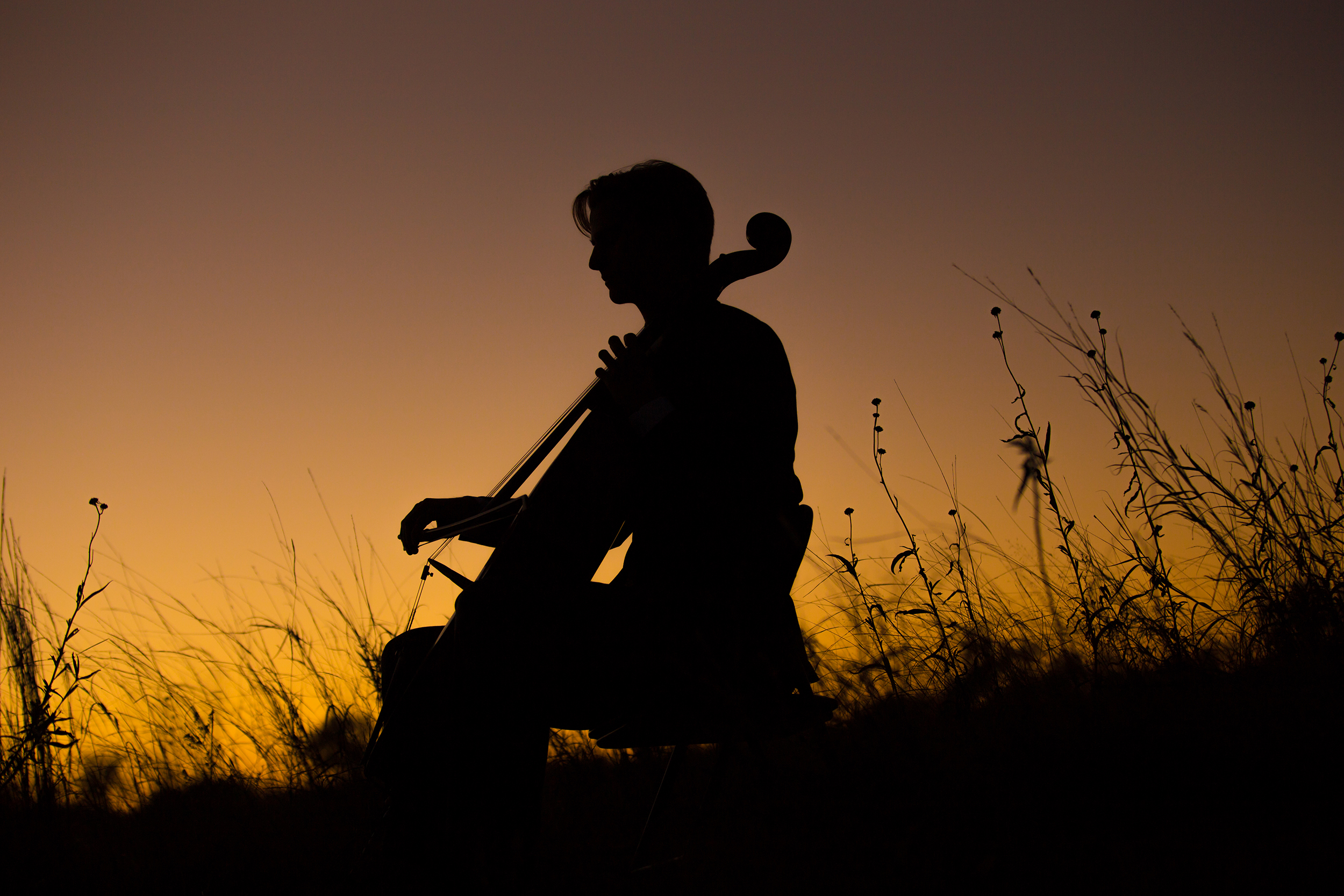In this artistically captured outdoor photograph set during the twilight hours, either at sunset or sunrise, a young man is seen in silhouette, playing a cello in the middle of a field. The photograph, almost square but slightly horizontally rectangular, shows him seated—likely on a chair, although it’s hard to distinguish due to the silhouette. His short hair is discernible only by shape as his features are enveloped in darkness. The sky, a gradient from a deep gray above to a glowing orange near the horizon, creates a striking backdrop without clouds. Surrounding the musician, numerous leafless plant stalks stretch upwards. The atmospheric yellowish hues towards the bottom of the image contrast with the stark silhouette, emphasizing the serene and solitary mood. No text accompanies the image, allowing the visual details to speak for themselves.